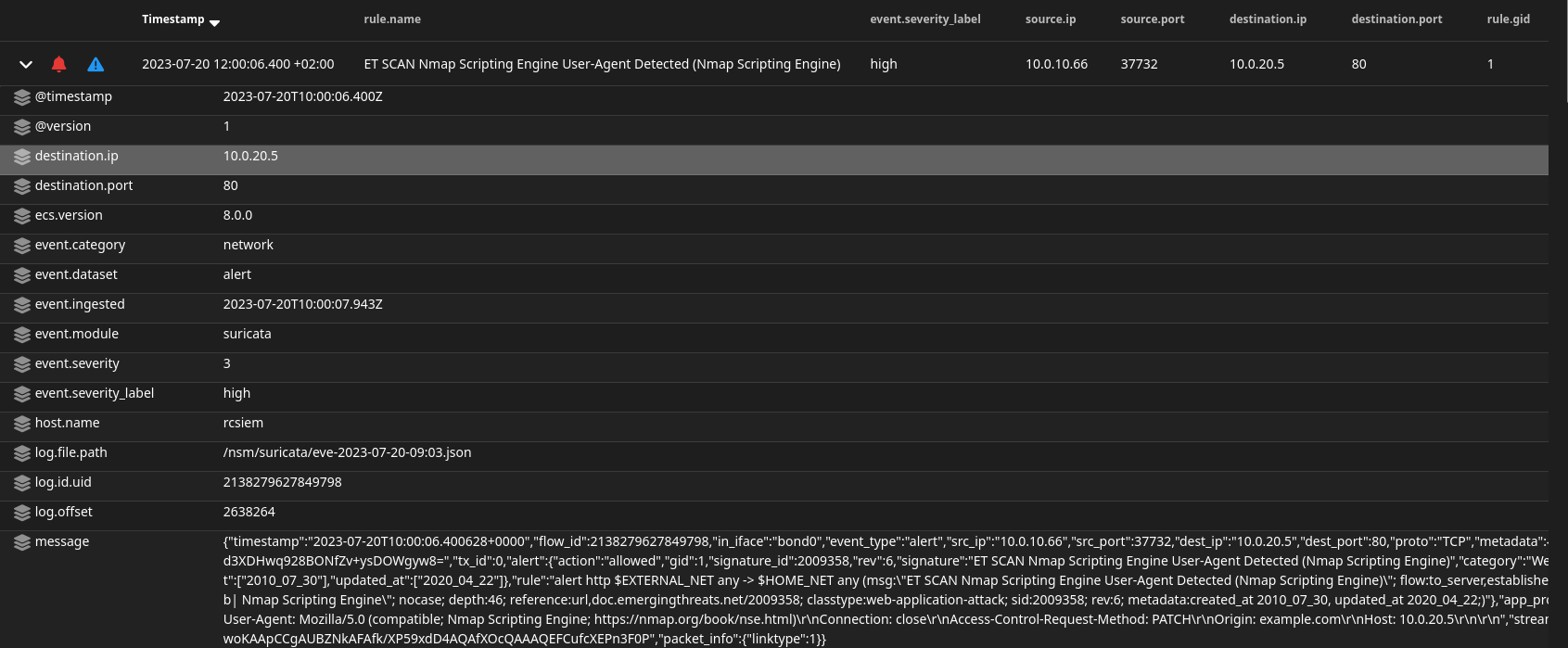This is an image of a dark-themed website or software interface. The background is composed of alternating shades of black and gray, giving it a striped appearance. Lines of text stand out in white font against the backdrop. On the left side, there appears to be a list of items, possibly files or directories, including an entry labeled "host.name." On the right side, there are columns or sections containing text with terms like "network" and "alert," along with a series of numbers. 

At the top left corner, there is a small red bell icon, typically indicative of notifications or alerts. Adjacent to this icon, slightly to the right, is a blue triangle with an exclamation mark inside, likely signaling a warning or important information. A white arrow pointing downward is located at the far left, possibly representing a dropdown menu or additional navigation options. 

Despite the detailed elements, the image is somewhat blurry, making it difficult to read the finer details clearly. The overall layout suggests an interface related to system monitoring or network management.